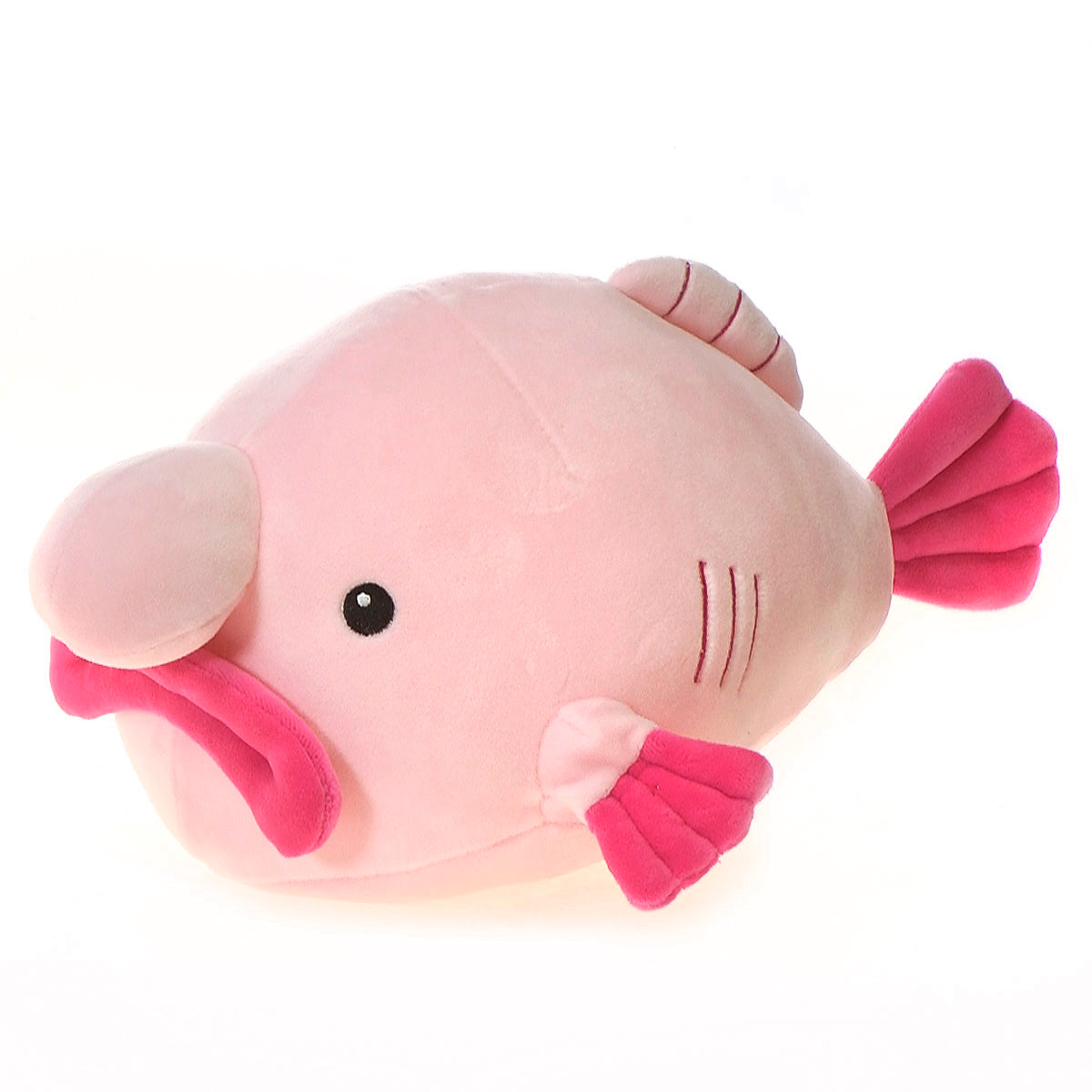This image showcases a whimsical and humorous plush toy modeled after the Viral Blobfish, a deep-sea creature known for its deflated appearance when brought to the surface. The plushie, however, appears rounded and significantly cuter, attempting to present a more attractive version of the blobfish. Positioned on a completely white background, the toy faces to the left, highlighting one small, beady black eye accented with a tiny white mark. The fish sports exaggerated, thick, darker pink, almost purple lips, which form a frown and give it a clown-like, sad expression. Its big, bulbous nose sits prominently above its lips, adding to its comical appearance. The plushie's body is a lighter pink, adorned with darker reddish pink accents and stripes, and features three gills just behind its side fin. Overall, the toy combines a human-like, clownish face with the odd body of a fish, evoking a sense of puffiness and endearing oddity.